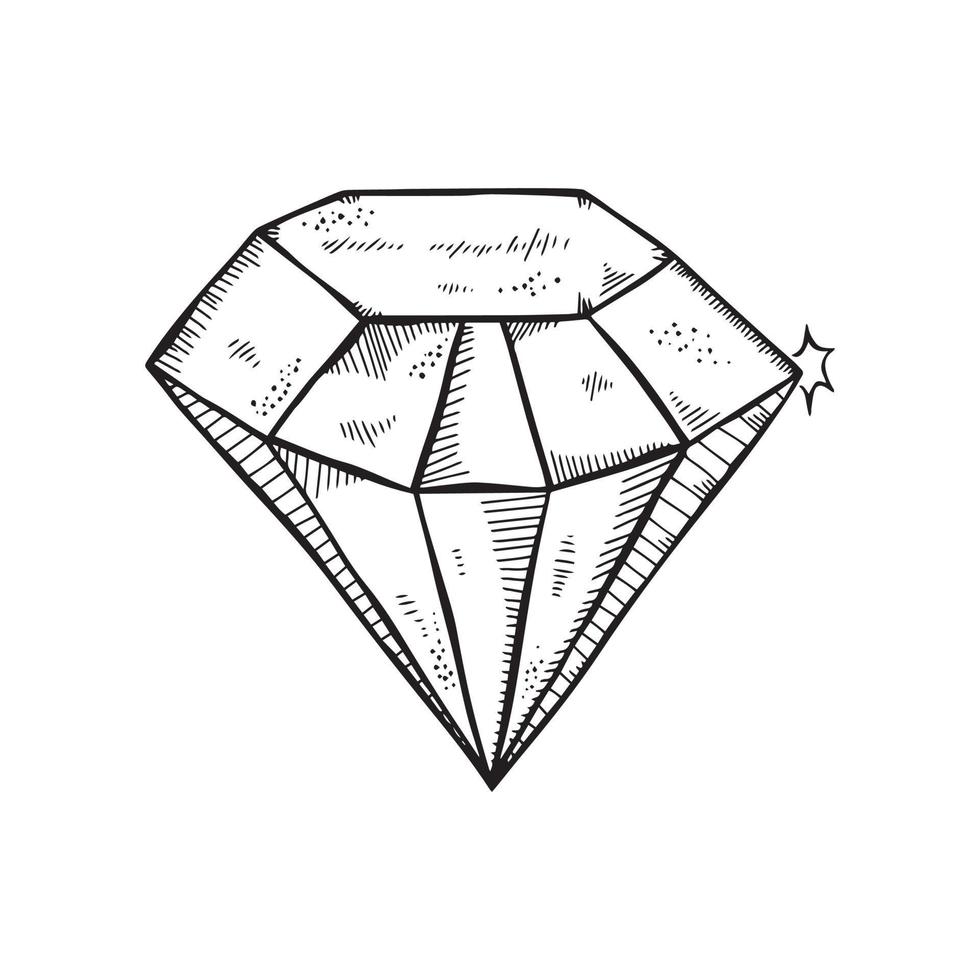This is a detailed black and white illustration of a diamond, drawn in ink. The diamond features a top that is flat, forming an octagonal or hexagonal shape, with a series of angled sections beneath it. Descending from the top, the diamond is sectioned into geometric facets, including several triangular forms that converge into a sharp point at the bottom. The drawing employs extensive use of cross-hatching, shading lines, and dots to indicate depth, three-dimensionality, and inclusions within the diamond. There is notable attention to the facets with horizontal and vertical lines, enhancing the perception of its intricate cuts. A small star symbol is drawn near the upper right-hand corner of the diamond, suggesting a sparkling effect. Additionally, some illegible writing or markings are present at the top, and the overall background remains white, emphasizing the detailed black ink artwork.